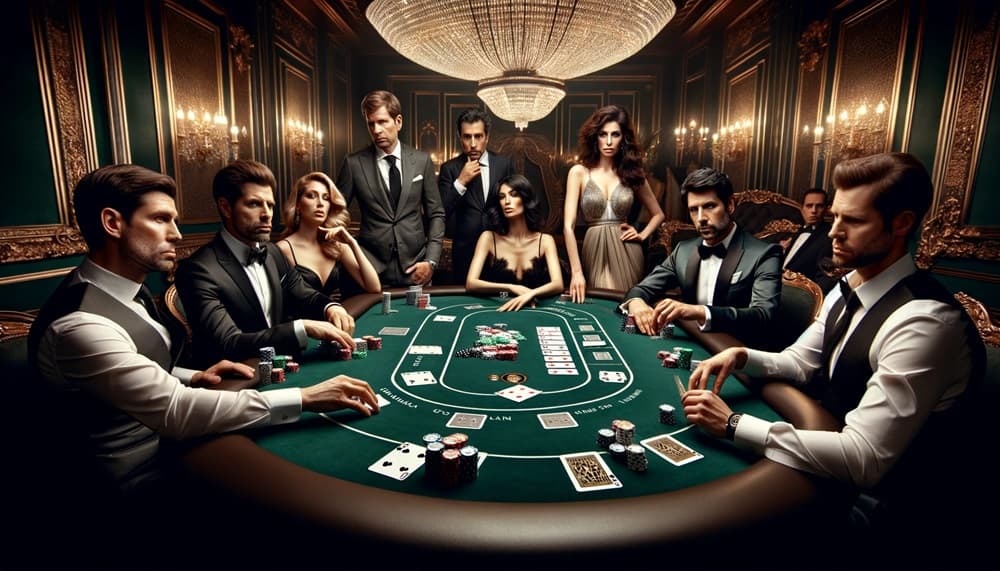The digital art illustration depicts a luxurious casino room centered around an oval-shaped poker table. The table itself features a rich green felt surface with a brown exterior and is adorned with playing cards and stacks of poker chips. Sitting around the table are four men in tuxedos and two women dressed in elegant black attire, all engrossed in the game with serious expressions and poker faces. 

Standing to the top right of the image is another woman, flanked by two men in suits behind a woman participating at the table. To the right side of the image, there is an additional man who appears to be observing the game rather than participating. The room's opulent ambiance is accentuated by golden-colored walls and a magnificent crystal chandelier with a smooth, dome-shaped design hanging prominently from the ceiling. The colors in the image range from blacks, tans, and browns to splashes of red, blue, and green, all contributing to the upscale and sophisticated atmosphere of the gambling scene.